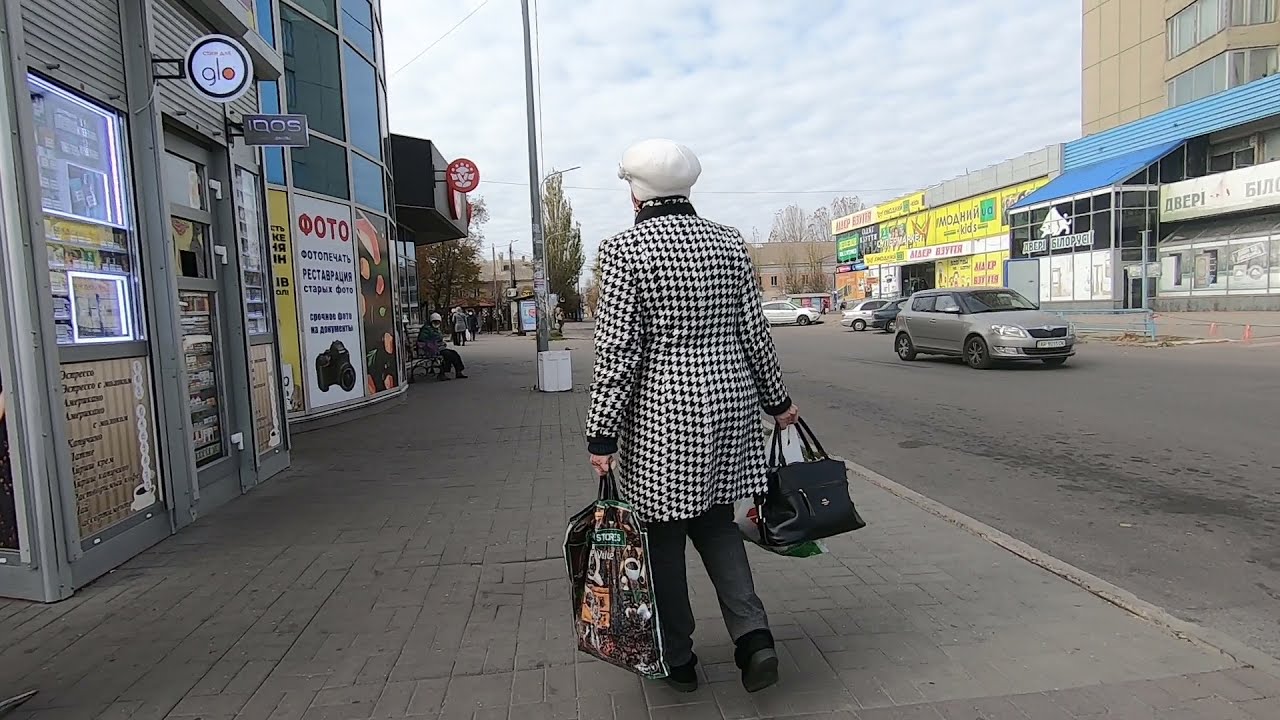In an urban setting under a mostly cloudy blue sky, a woman is seen walking across a sidewalk. She is in the center of the image, wearing a distinctive white and black patterned jacket with a black collar and a white cap. Her gray pants and black shoes with gray bottoms complement her attire. The woman carries a black purse and a white plastic shopping bag in her right hand, while her left hand holds a shopping bag adorned with pictures of coffee and coffee cups. To her left, various storefronts with neon lights and gray paneling line the street, their displays reflecting off the windows. On the right side of the image, a gray asphalt road stretches out with no markings, occupied by a silver van and a few more scattered cars in the background. A yellow building, a structure with a blue canopy, and a tan building add to the urban backdrop, making the scene appear bustling yet composed.